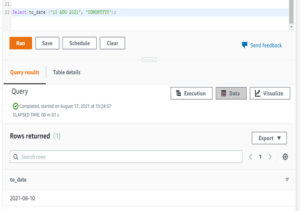The image depicts a detailed snapshot of a web-based code editor interface. At the top of the page, there is syntax-highlighted code featuring segments in purple, black, and green colors, all presented against a blue-highlighted background with the line number "22" beside it. Beneath this code, an orange "RUN" button is prominently displayed alongside options to "Save," "Schedule," and "Clear." Additionally, a blue "Send Feedback" button is visible, likely meant for user suggestions or bug reports.

Below the code section, the interface includes a "Query Results" area with a status message stating "Query Completed." It notes that the query started on August 17th, 2021, accompanied by a timestamp. This area is supplemented with various functional buttons labeled "Execution," "Data," and "Visualize," facilitating different modes of output analysis.

Further down, there is another section titled "Rows Returned," featuring a text box for input or display purposes and an "Export" button for data extraction. The interface also includes multiple search fields to filter results.

The overall background of the interface is predominantly gray. It contains additional black-text buttons offering various configuration and navigation options. A gray gear icon suggests access to settings, and the layout implies that users can navigate through different pages, likely within the same web application. The design and functional elements give the impression of a versatile, interactive code and data management platform, enabling users to execute, visualize, and manipulate queries efficiently.